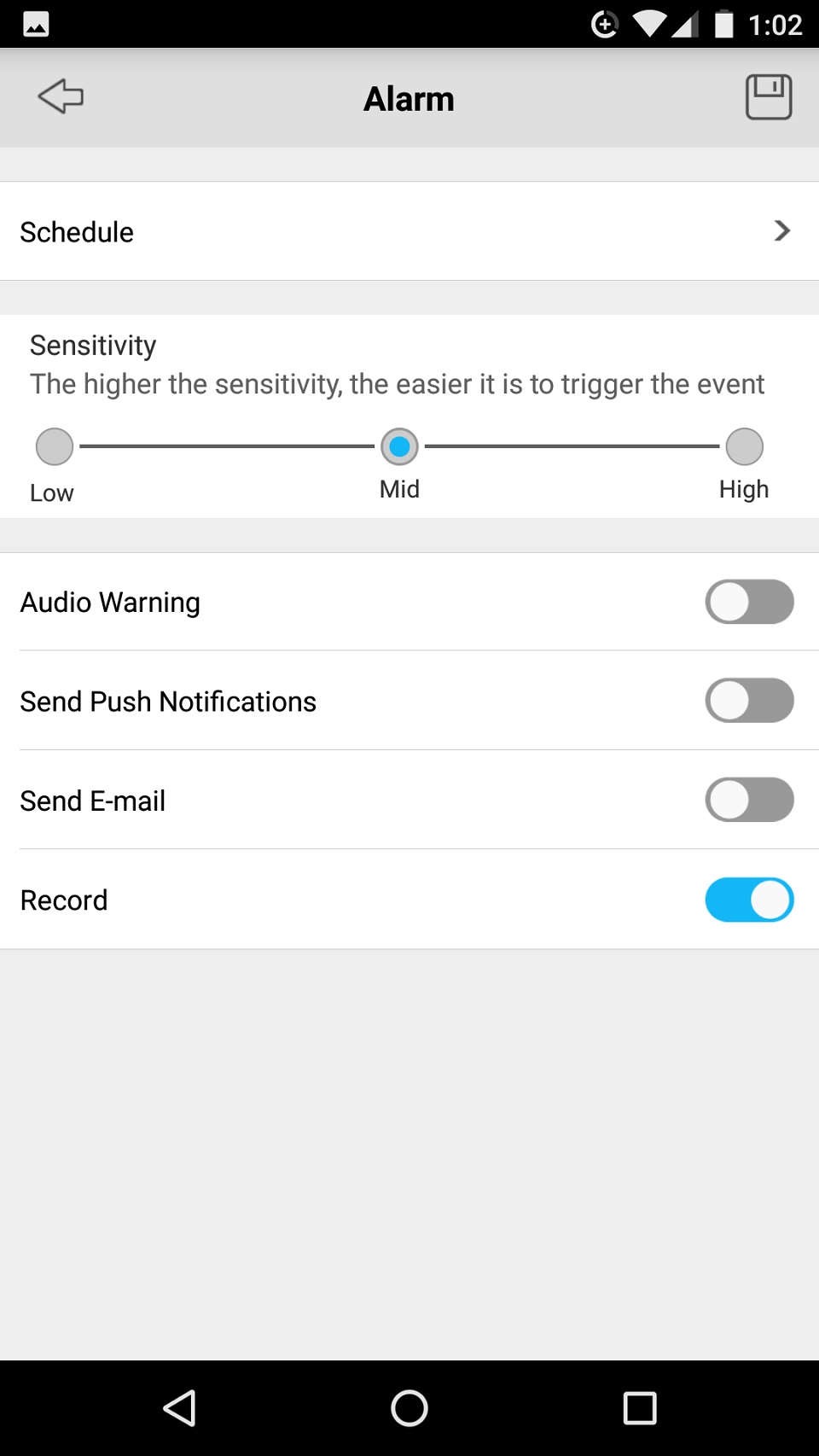### Caption

The image showcases an Android device's alarm scheduling settings, possibly for either a phone or a tablet. The interface is displayed against a backdrop with black banners at the top and bottom, while the central panel features a mix of grey, white, aqua blue, and black colors. 

At the top of the screen, the status bar reveals essential elements: Wi-Fi signal, cellular bars indicating three bars of reception, and a battery icon showing a full charge. The time displayed is 1:02 PM. Additionally, there is a small icon resembling an old-fashioned floppy disk in the upper right-hand corner, suggesting the presence of file-related features or actions, along with a directional arrow.

Key details from the settings include a "Schedule Sensitivity" option set to "mild", indicating a moderate threshold for triggering the scheduled event. Below this, various notification preferences are displayed: "Audio Warning" is turned off, "Send Push Notifications" is turned off, and "Send Email" is also turned off. However, the "Record" button is activated. Despite the interface suggesting alarm functionality, the exact application or purpose of this alarm remains unclear.